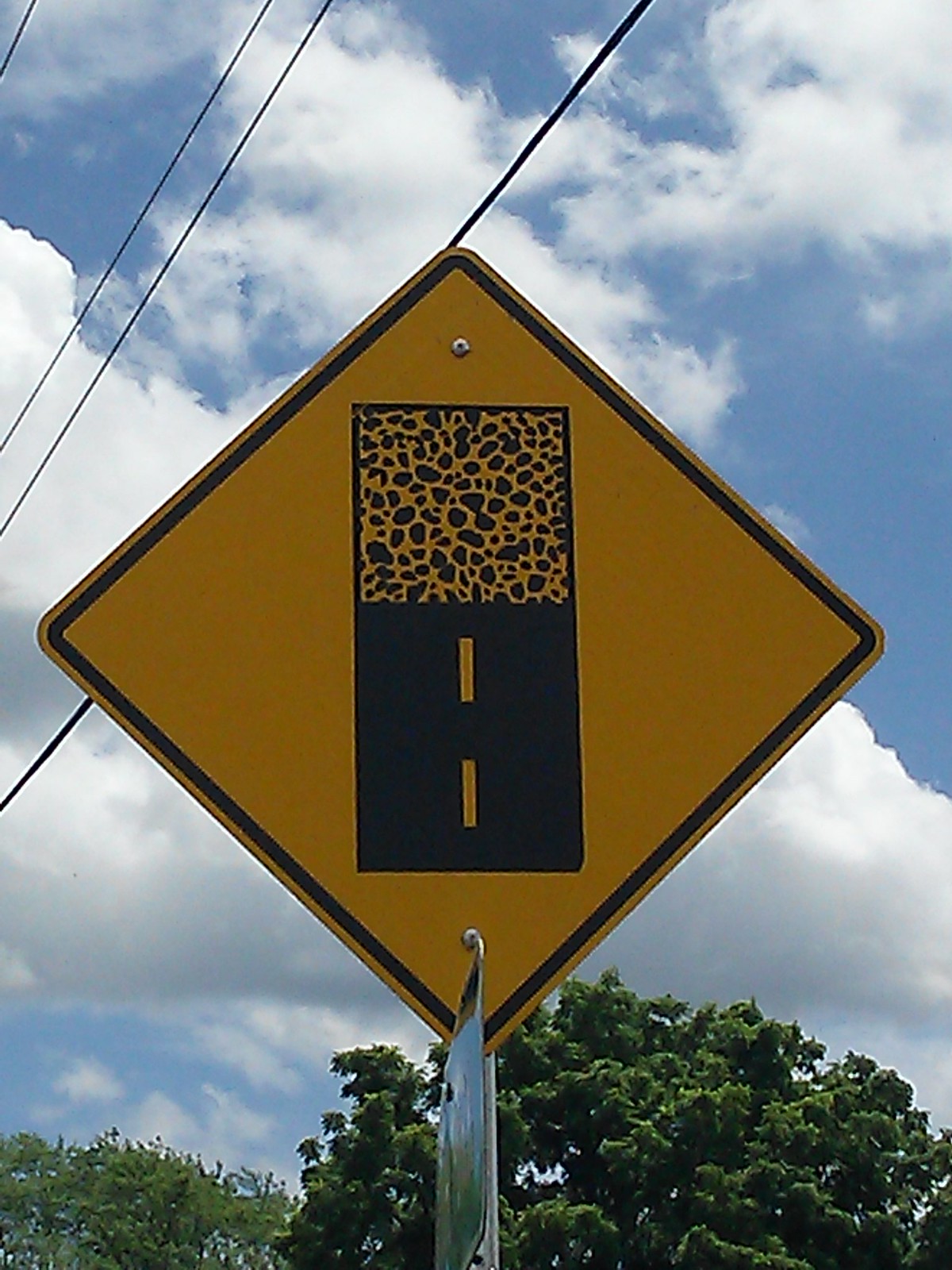A vivid photograph showcasing a distinctive yellow diamond-shaped road traffic sign bordered in black is the focus of this image. The sign, prominently displayed against a backdrop of clear blue skies accented with puffy white clouds, stands out amidst the surrounding natural greenery of trees adorned with lush green leaves. The sign itself is divided into two halves: the bottom half features a depiction of a paved road with two yellow dividing lines, symbolizing a conventional roadway. The top half shows a transition into a gravel or unpaved surface, suggesting an upcoming change to a more rural or remote road. The sign is affixed with two visible nuts, one at the top and one at the bottom, and is accompanied by a few overhead wires that traverse the sky. The overall composition captures a moment of serene, sunny weather in a seemingly tranquil area.